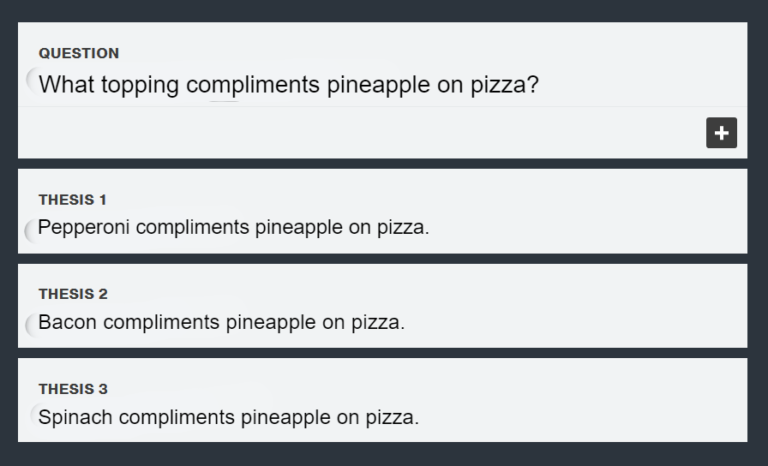This image features a structured grid layout consisting of four rows, each contained within a clearly defined white box outlined in black. The largest box, titled "Question," is prominently positioned at the top and occupies the most space. Its white background centers the query, "What topping complements pineapple on pizza?" with a black plus sign situated in the bottom right corner.

Below this, three equally-sized boxes are aligned in a single row, each bearing a different proposition regarding pineapple pizza toppings. The first box, labeled "Thesis 1," asserts "Pepperoni complements pineapple on pizza." Adjacent to it, the second box, "Thesis 2," states "Bacon complements pineapple on pizza." The final box, "Thesis 3," claims "Spinach complements pineapple on pizza." The uniform spacing between the boxes ensures a balanced and symmetrical appearance. All the text within the boxes is black, providing a stark contrast against the white background, enhancing readability and visual clarity.